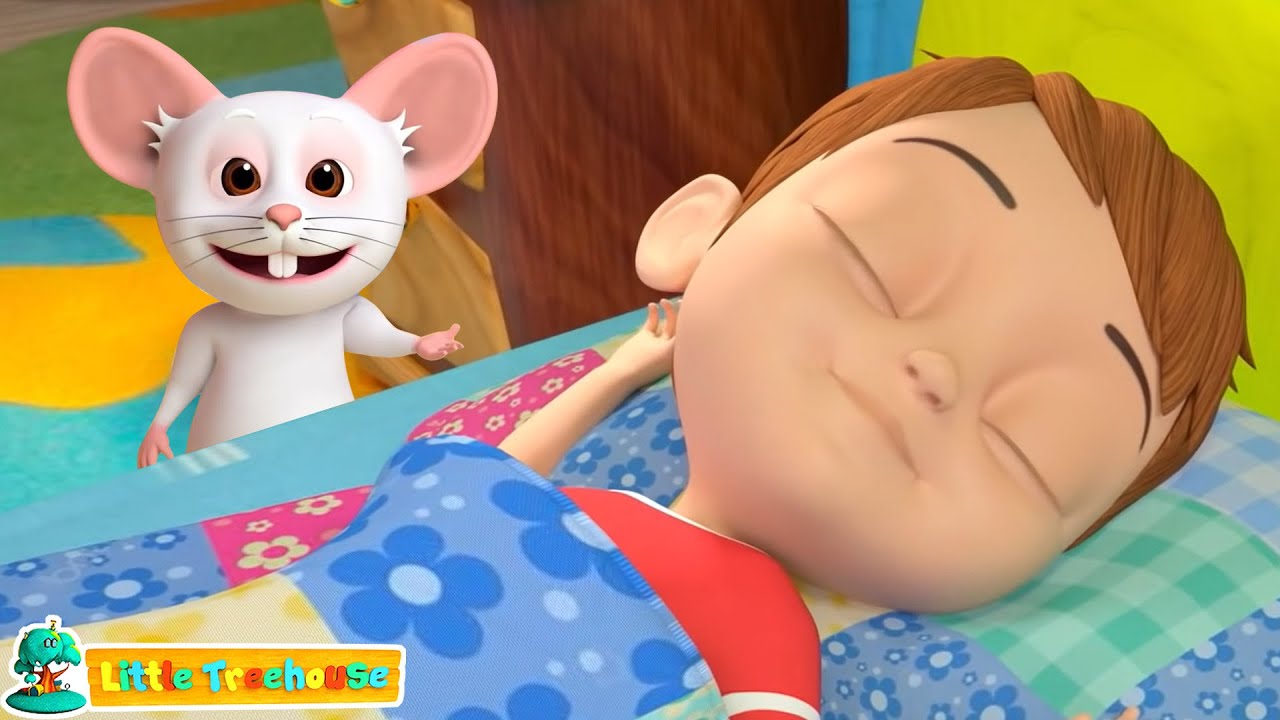This image appears to be a still shot from a low-budget, computer-generated children's cartoon, likely part of an educational show. The setting is a cozy bedroom where a young boy with brown hair and large ears is soundly asleep on a blue bed. He is wearing a red shirt with white trim and lies on a multicolored gingham-checked pillow, his head turned towards the viewer. He is covered by a floral-patterned comforter featuring blue, yellow, and pink squares. In the top right corner of the image, a cheerful white mouse with oversized pink ears, brown eyes, a pink nose, and two prominent buck teeth stands with his pink hand outstretched, smiling at the camera. The headboard behind the boy is yellow and blue, and the bed is accompanied by a teal, yellow, and green geometric rug and a brown dresser. Adding to the whimsical charm, the bottom left corner of the image features a colorful graphic that reads "Little Tree House" in various shades of yellow, green, blue, and red letters, next to a cartoon treehouse, depicted on a circular patch of grass.